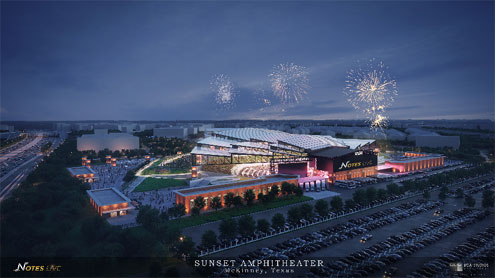The image is an advertisement featuring an aerial nighttime view of the Sunset Amphitheater, as indicated by the text at the bottom of the picture. The primary focus of the image is a large, well-lit amphitheater displaying vibrant purple and pink lights, surrounded by several smaller buildings. In the dark, muted blue and gray sky above, fireworks are bursting, adding a festive atmosphere. On the left side of the image, a busy highway can be seen, and in the lower right-hand corner, there's a large parking lot filled with numerous cars, alongside rows of trees. The image conveys a sense of a lively event with numerous attendees, highlighted by the many cars parked around and the celebratory fireworks overhead.